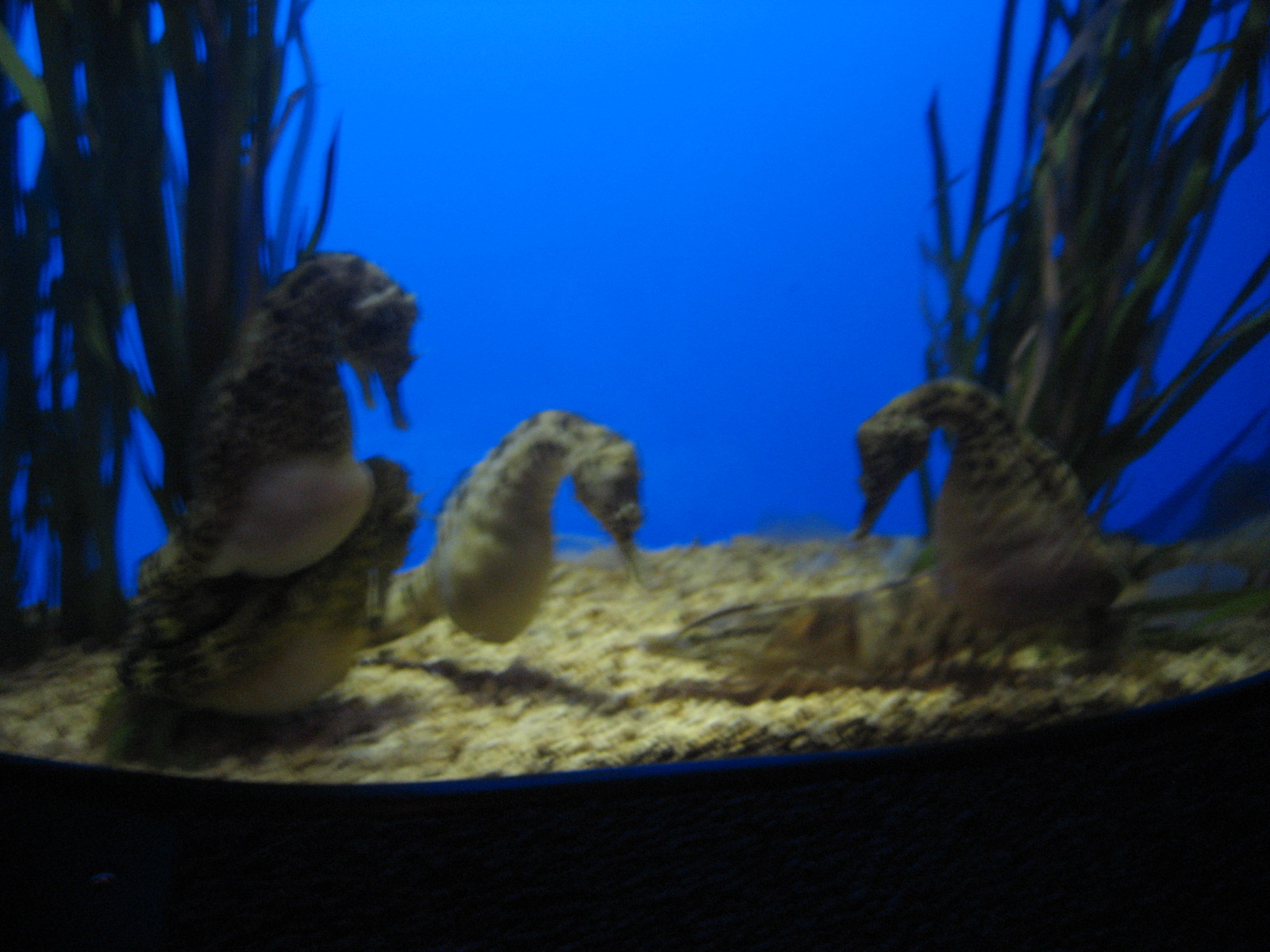This image, taken in an aquarium, depicts a vibrant scene dominated by a striking electric blue background. At the bottom of the aquarium, there is a substrate of yellowish gravel or thick sand, upon which tall, thin-leaved plant life rises upward, resembling greenish grass or seaweed. The focus of the image is on several large seahorses with rounded bodies and necks, scaly skin, and dark brown coloration with darker striping. There are four seahorses in total, though the photograph is somewhat blurry. The two on the left are stacked one above the other, the one in the middle is illuminated by the light above, casting it in a yellowish-tan hue, and the one on the far right is more shadowed. All the seahorses have pronounced, bulging bellies, suggesting they may be pregnant males. There is also a small fish present in the scene, much smaller than the seahorses, adding to the dynamic underwater environment.